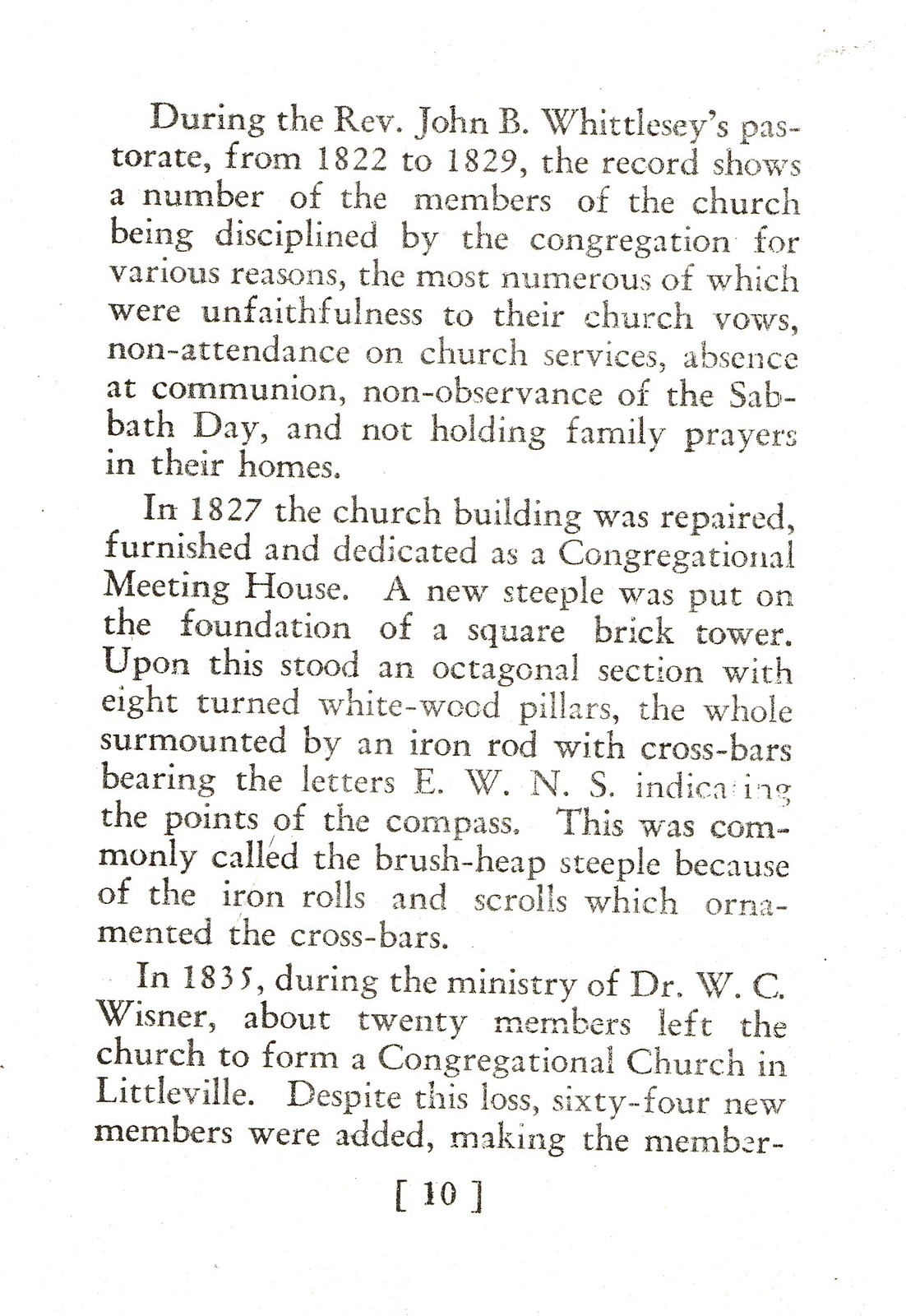The image depicts a scanned page from an old book, showcasing black text on a white background. The passage details historical events from a church's history during the Rev. John B. Whitley's pastorate from 1822 to 1829. The church disciplined members for various transgressions, including unfaithfulness to church vows, non-attendance at services, absence at communion, non-observance of the Sabbath, and failure to hold family prayers. In 1827, the church was repaired and dedicated as a congregational meeting house, featuring a new steeple atop a square brick tower with an octagonal section supported by eight white wood pillars, and an iron rod with crossbars inscribed with the compass points E.W.N.S., known as the Brush Heap Steeple due to its ornate iron rolls and scrolls. The text also mentions that in 1835, under Dr. W.C. Wisner's ministry, 20 members left to form a new church in Littleville, but 64 new members joined despite this loss. The passage cuts off mid-sentence, resuming on the following page. For more information, visit www.fema.gov.